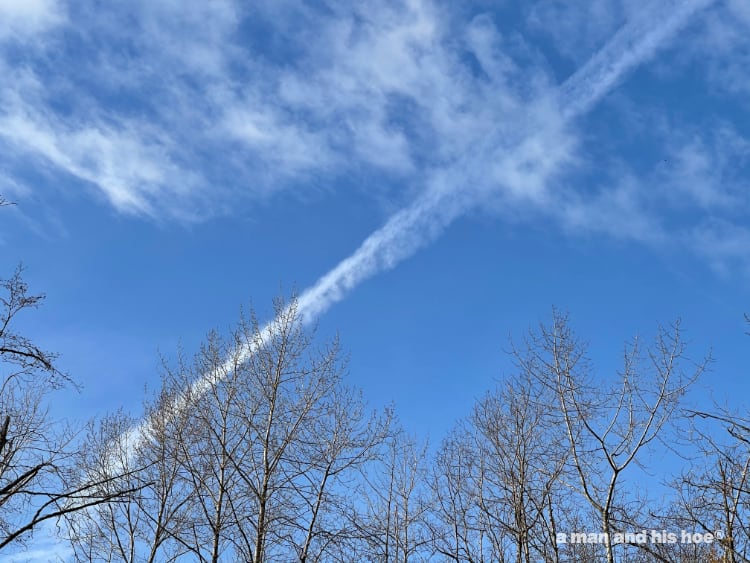The photograph captures a striking upward view towards a brilliant blue sky, featuring a gradient from dark to light blue near the top of the image. Wispy clouds meander across the heavens, with a distinct jet stream cloud slicing diagonally from the upper right to the lower left. The scene is framed by the dark, barren treetops of several leafless trees, suggesting a late fall or early winter setting. The absence of any foliage highlights the stark contrast between the silhouetted branches and the vibrant sky. In the lower right-hand corner, partially transparent white text reads, "a man and his hoe," followed by a small copyright symbol.